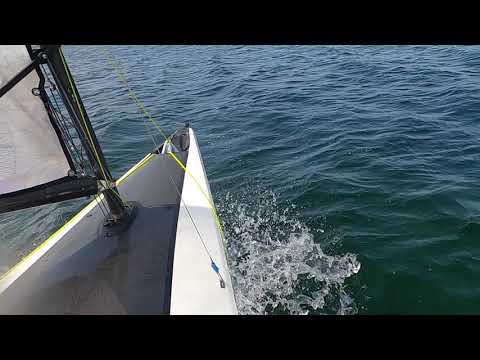The image, taken from the point of view of someone who is windsurfing, showcases a windsurfer cutting through mostly dark green water. The water surrounding the windsurf board is slightly choppy, creating white splashes where the board slices through. The windsurf board itself is distinctively triangular, with white edges and a central gray section. Emerging from the center of the board, the sail features a black mast and a white canvas adorned with black trimming. A network of bright yellow wires and ropes connects the board to the mast, adding vibrant, neon highlights to the scene. There’s a notable small cubby located near the front nose of the board. The sail is fully extended, emphasizing the motion and dynamic nature of the windsurfing experience.